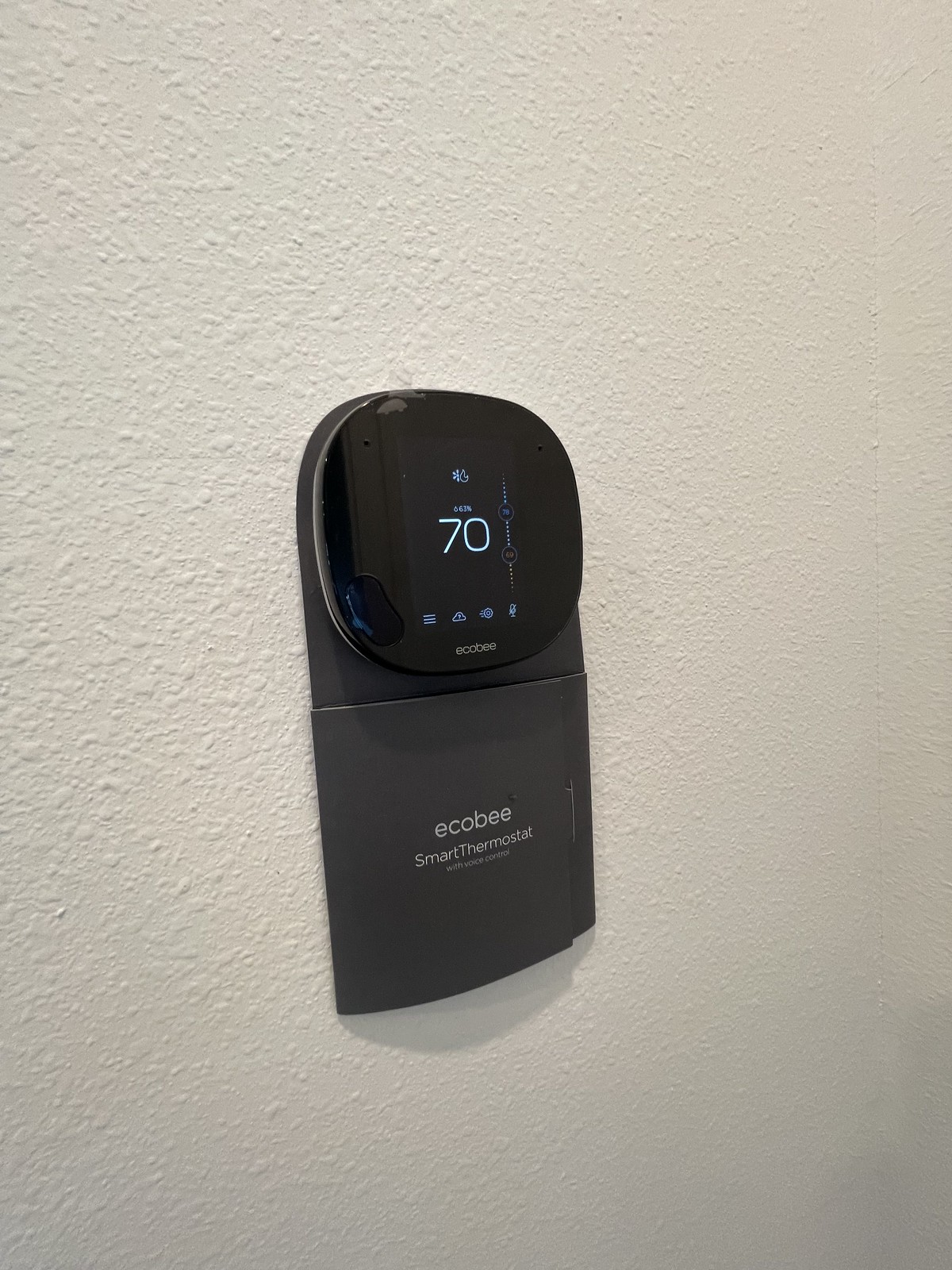This photograph showcases an Ecobee Smart Thermostat, stylishly mounted on a white concrete wall. The thermostat features a sleek, slightly gray rectangular frame with a rounded top, housing a glossy black display that exudes modernity. 

Central to the display is a prominent white numeral '70,' indicating the current temperature. Positioned just above this, there is a water drop icon followed by the humidity level, '63%'. 

Further up, an icon resembling half of a sun or a flower accompanies a wavy line, likely symbolizing the thermostat's current mode. To the right of the temperature reading, a series of dots spans vertically from a blue circle marked '78' at the top, to a red circle labeled '68' at the bottom, with intermediate dots shaded in orange, illustrating a temperature range or schedule. 

At the display's bottom, several icons are neatly arranged: a hamburger menu icon, a cloud icon, a gear icon, and a microphone icon with a strikethrough, providing various functional shortcuts.

Overall, the Ecobee Smart Thermostat merges functionality with elegant design, standing out against the serene backdrop of the wall it's affixed to.